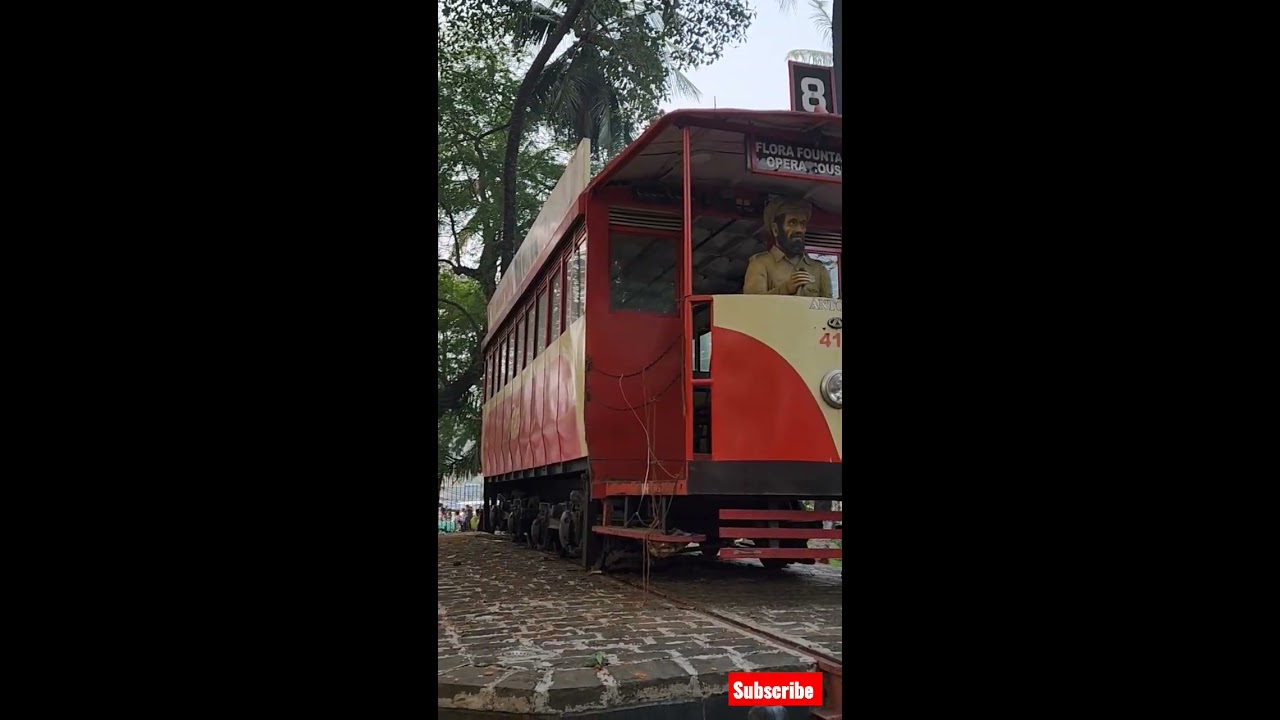In this detailed outdoor image, we see a red tram or trolley car stationed on a cobblestone pathway, likely serving as a display piece rather than an operational vehicle. The tram features beige or tan outlines detailing its body, and at the front top, a black sign prominently displays the number 8. Below this sign, partially visible text reads "Flora Fountain Operations." Inside the tram, situated to the right, is a highly realistic mannequin or statue of a bearded man with a brown turban and matching brown shirt, likely representing an Indian or Sikh individual. This figure adds a touch of historical or cultural context to the display. The tram’s design also includes a partially obscured headlight and the numbers 4 and 1 in red on either side, hinting at its route or identification. Adjacent to the tram are stairs leading up into it. The surrounding area features dark brown brick-style paving, and in the background, lush green trees are visible against an open sky. The foreground includes a red box with the word "Subscribe" written in white, and both sides of the image are bordered by black.